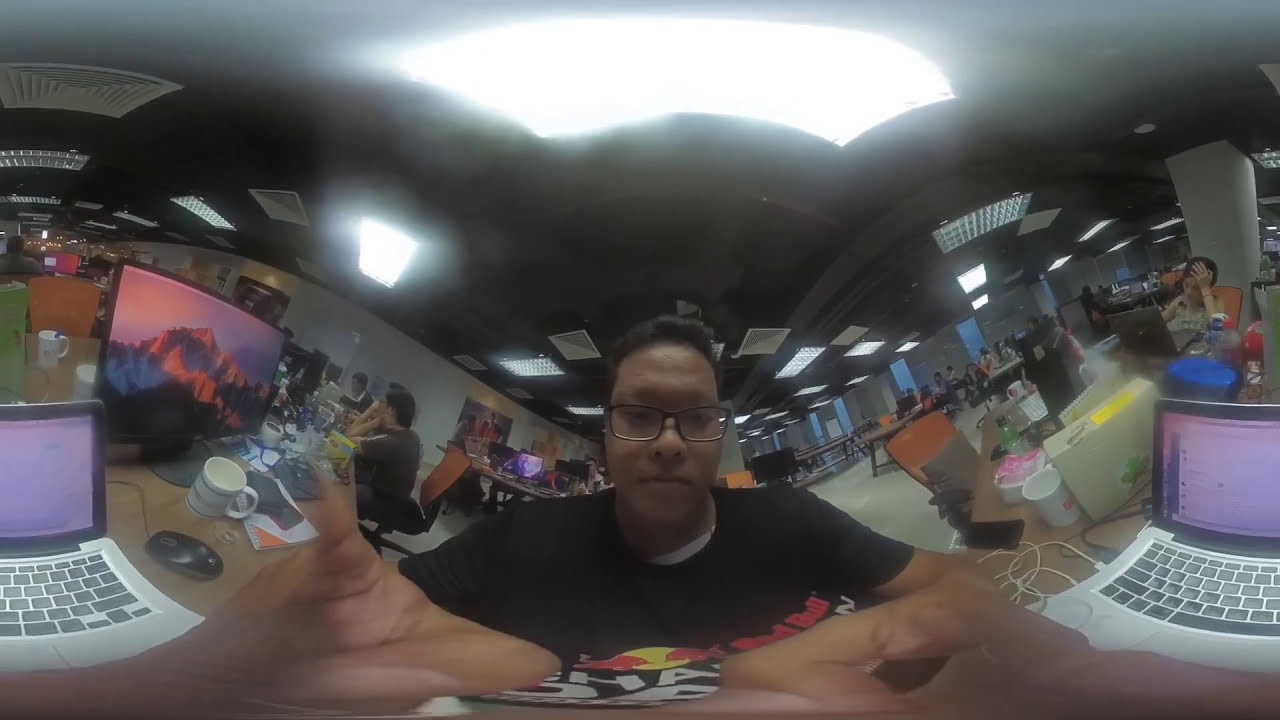This is an indoor photograph seemingly taken through a fisheye lens, displaying notable curvature and distortion. The focus is a close-up, albeit blurry, of a young, medium-complexioned man seated at a computer workstation, facing the camera. He appears to be in motion, with his outstretched hands visible near the bottom edge of the image, making it unclear what he's handling. He wears a black t-shirt featuring a Red Bull logo, with a white shirt peeking out from underneath. His short dark hair frames his face, which is adorned with dark-framed glasses and a wide nose, possibly exaggerated by the blurred focus. 

The background reveals a busy office environment with fluorescent ceiling lights, various tables, and multiple occupied desks. To the man's right and left, there are computers, including a laptop and a monitor. Further back, several colleagues, many of whom appear to be Asian, are visible at their workstations, working diligently with computers and other office equipment. The whitish walls and scattered coffee mugs emphasize the bustling, professional ambiance of the space.